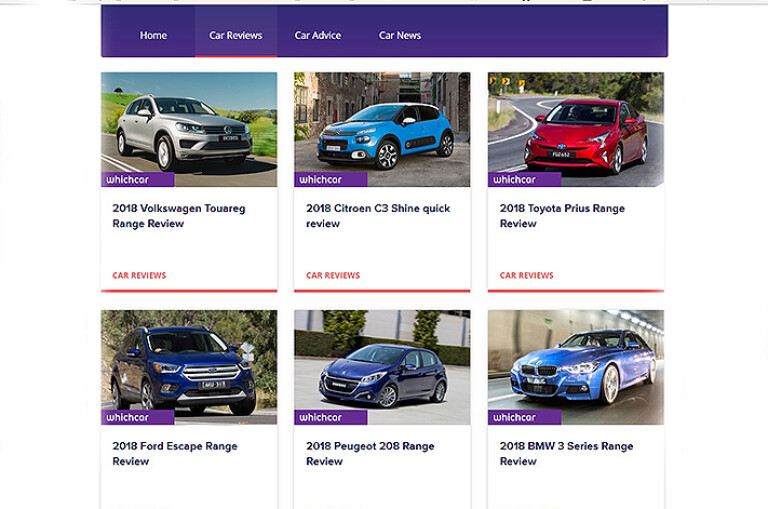The image is a feature page from a car review website, characterized by a clean, structured layout. The header has a rich purple background with navigation tabs written in white. The tabs include "Home," "Car Reviews," "Car Advice," and "Car News." The "Car Reviews" tab is highlighted with a red underline, indicating it as the active section.

Beneath the header, the main section features a collage of six car images, each accompanied by descriptive text. All text overlays follow a consistent style with white letters against a purple backdrop, clearly stating "Which Car" over each vehicle.

1. **Top Left**: The image shows a silver-grey 2018 Volkswagen Touareg. The caption reads, "2018 Volkswagen Touareg Range Review," with "Car Reviews" in orange text at the bottom. The model name is emphasized in black text on a white background.

2. **Top Center**: Here we see a blue 2018 Citroën Cedric Shine with a notable white rooftop. The caption reads, "2018 Citroën Cedric Shine Quick Review."

3. **Top Right**: This spot features a fiery red 2018 Toyota Prius. The caption identifies it as the "2018 Toyota Prius Range Review."

4. **Bottom Left**: The image presents a blue Ford Escape, captioned as "Ford Escape Range Review."

5. **Bottom Center**: Displayed in this image is another blue vehicle, identified as the "2018 Peugeot 208 Range Review."

6. **Bottom Right**: The final image shows a blue 2018 BMW 3 Series traveling through a tunnel illuminated by lights. The text reads, "2018 BMW 3 Series Range Review."

Each car image is carefully labeled, ensuring readers receive detailed information at a glance, enhancing the user experience on the review page.